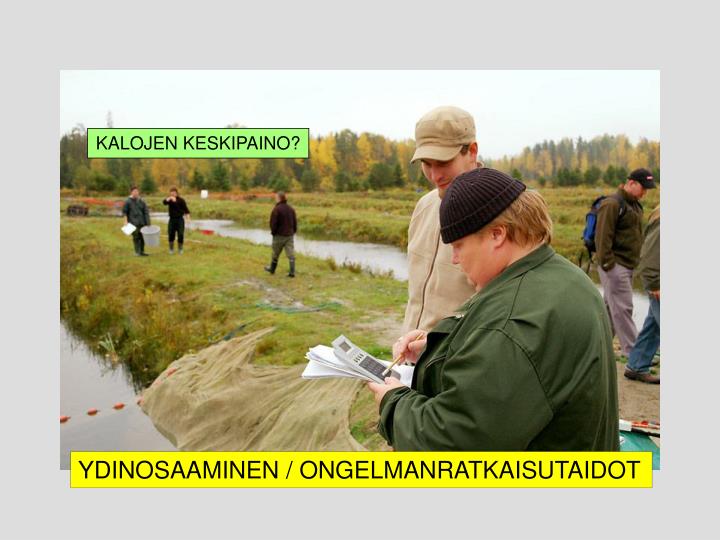In this photograph with a plain gray border, a scene unfolds with seven individuals situated in a grassy field by a little creek or irrigation ditch. The setting appears to be farmland, bordered by two bodies of water. In the foreground, a somewhat larger man in an olive green shirt and black knit cap is focused on a stack of papers in his hand, using a pencil in his right hand to guide a second man, who stands to his right. This second man is dressed in a beige jacket and matching baseball cap. Together, they seem engaged in a discussion about the documents.

In the background, five people are dispersed across the grassy terrain. On the left, a person holding a large white bucket and another clipboard is seen in dark attire with large rubber boots. Near the center-left, a man in a green sweatshirt, blue backpack, black hat, and gray pants stands nearby another individual in a greenish-colored coat and blue jeans. Further back, on the right, a man in a brown shirt and green pants equipped with flood boots walks alone. A dense forest frames the scene in the far background.

The image contains captions in a foreign language. A green band in the upper left corner displays non-English text, potentially reading "Kelegan Kespupeno?" Meanwhile, at the bottom of the foreground, a yellow band features additional non-English text, faintly deciphered as "You’re just a nun some men are men/angle men tray case who they don’t."

Overall, the image captures a moment of interaction and activity among the individuals on this stretch of grassland, with their varied attire and tasks indicating a possible outdoor or agricultural endeavor.